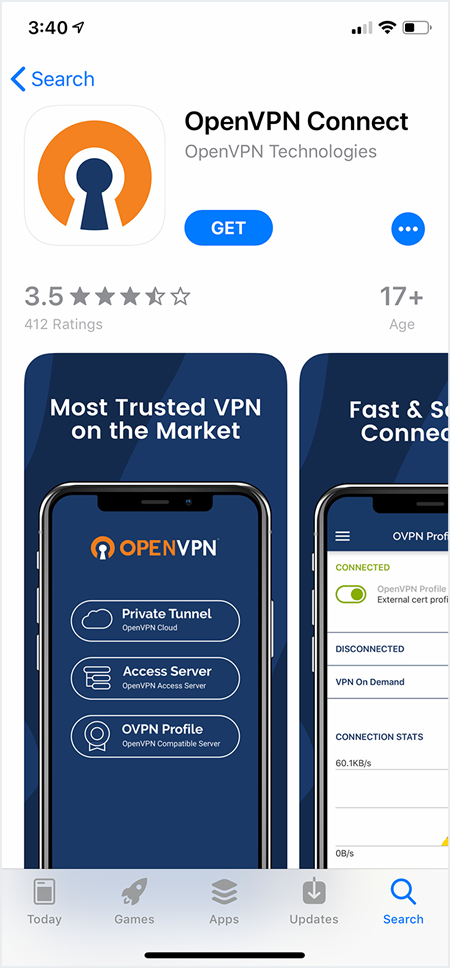This image captures a screenshot of a mobile device displaying the iOS App Store interface. At the very top left corner, the time is shown as 3:40. In the top right corner, the status indicators are visible, including a full network signal bar, a WiFi signal strength indicator showing 3 out of 3 bars, and a battery level icon indicating a nearly full charge.

The main body of the screenshot highlights search results for the term "open VPN." Various app descriptions and names can be seen, including "OpenVPN Connect," "OpenVPN Technologies," "Most Trusted VPN on the Market," "Private Tunnel," "Access Server," and "OVPN Profile."

Below these search results, several category tabs are visible, including "Today," "Games," "Apps," "Updates," and "Search," confirming that this is indeed the iOS App Store. The overall layout and interface features further reinforce that this screenshot is taken from an iOS device.